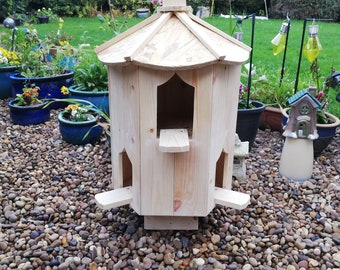The photograph depicts a charming garden scene featuring a central wooden birdhouse, resting on a bed of multicolored river rock pebbles. The birdhouse, likely crafted from unfinished plywood, has a unique six-sided design with a triangular sloping roof and three windows arranged in alternating heights on each face. Flanking the birdhouse are a variety of blue and reddish pots brimming with vibrant flowers in shades of yellow, green, and orange. Surrounding the scene is a lush, well-maintained green grass lawn, with additional garden decorations adding to the delightful setup. In the distant background, hedges, bushes, and trees can be seen, completing the picturesque outdoor space.